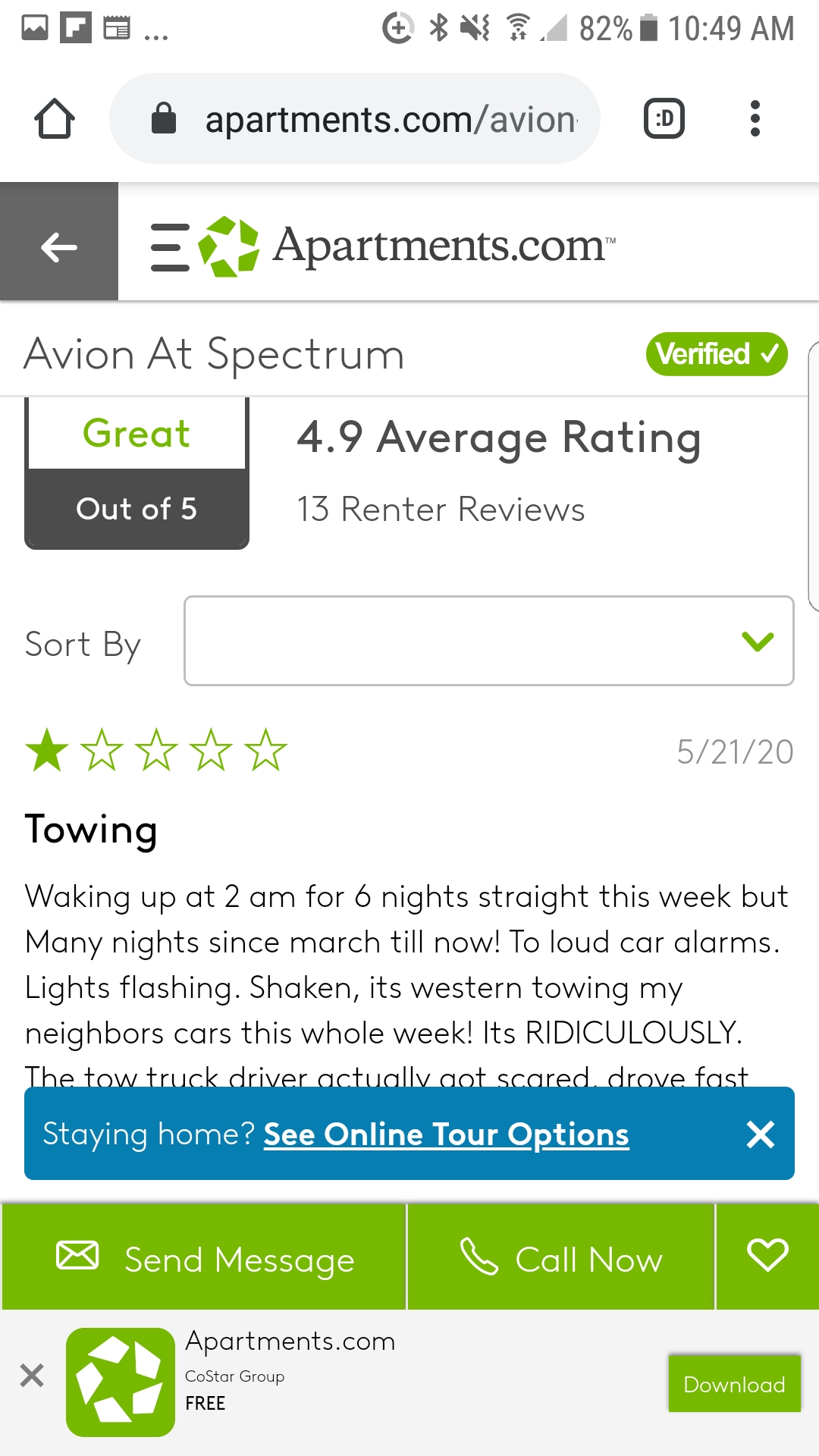Certainly! Here's a cleaned-up and detailed caption:

---

The image is a screenshot taken on a smartphone from the Apartments.com website. The screenshot features a white background throughout. In the top left-hand corner, there are several app notifications, although the specific apps are not discernible. On the top right-hand side, indicators for time, battery percent, battery icon, service signal strength, Wi-Fi, Bluetooth, battery saver, and audio are visible.

Below these indicators is the web address bar displaying "apartments.com/avion," though part of it is cut off. A tabs bar and a home menu are also present beneath the address bar. Further down, the Apartments.com logo and a navigation bar with a back button are visible.

The main content starts with the title "Avion at Spectrum." Next to the title, in a white font on a green background, is a verification label reading "Verified." Below this, a rating of "4.9" out of 5 is displayed, based on 13 renters' reviews. A grayed-out "Sort" option is also available.

The screenshot includes a highlighted portion of a one-star review dated 05-21-20. The review mentions disturbances caused by towing activities: "Waking up at 2 a.m. for six nights straight this week, but many nights since March until now. Too loud car alarms. Lights flashing. Shaken. It's western towing my neighbor's cars this whole week. It's ridiculously..." Unfortunately, the review text is partially obscured by a pop-up notification.

The pop-up notification, with white text on a blue background, reads "Staying home? See online tour options." Below this, there are buttons labeled "Send Message," "Call Now," and an icon of a heart for favoriting the listing. There's also an option to download the Apartments.com app.

---

This caption provides a comprehensive and detailed description of the screenshot contents.